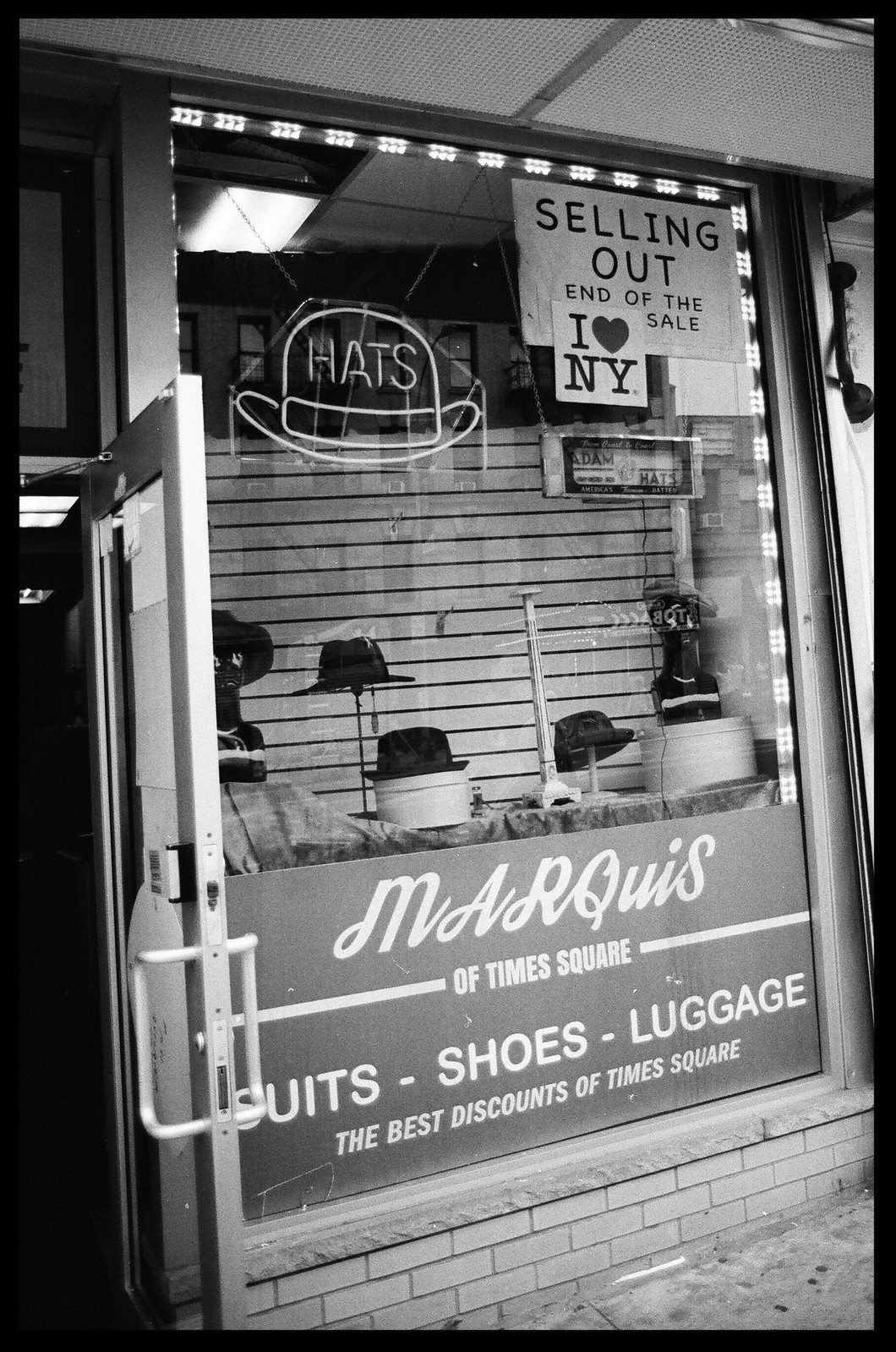This black-and-white photograph captures the front of a hat shop located outdoors, showcasing a classic scene with a plate glass window. Behind the window, five hats—featuring a mix of derbies and fedoras—are elegantly displayed on hat stands against a backdrop of Venetian blinds. A prominent neon sign reading "HATS" shines above, accompanied by a sticker proclaiming "I Love New York." Beneath the hats, a sign declares "Selling Out. End of the Sale." The window itself bears the name "Marquis of Times Square" in bold letters, with additional signage below advertising "Suits, Shoes, Luggage" and "The Best Discounts of Times Square." To the left of this display, a plate glass door stands open, inviting passersby into the store where fluorescent lights illuminate the interior. In front of the shop, a low brick wall and sidewalk complete the composition of this nostalgic scene in New York City’s bustling Times Square.